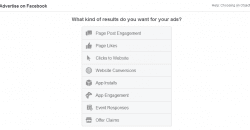A screenshot displays a Facebook advertising interface. Starting from the top left, the bold black text "Advertise on Facebook" stands out. Moving rightwards, there is a faint and blurry string of letters and numbers, resembling a code. Below this, a light gray line spans the width of the screen. Centered beneath the line, bold black text reads "What kind of results do you want for your ads?" Immediately below, a light gray rectangular area contains eight smaller, vertically-stacked rectangles forming a larger vertical column. Each smaller rectangle is separated by faint gray lines. On the left side of each rectangle, an icon is displayed, while the corresponding description is on the right. The descriptions from top to bottom are: "Page Point Engagement," "Page Likes," "Clicks to Website," "Website Conversions," "Age and Gender," "App Engagement," "Event Responses," and "Other."